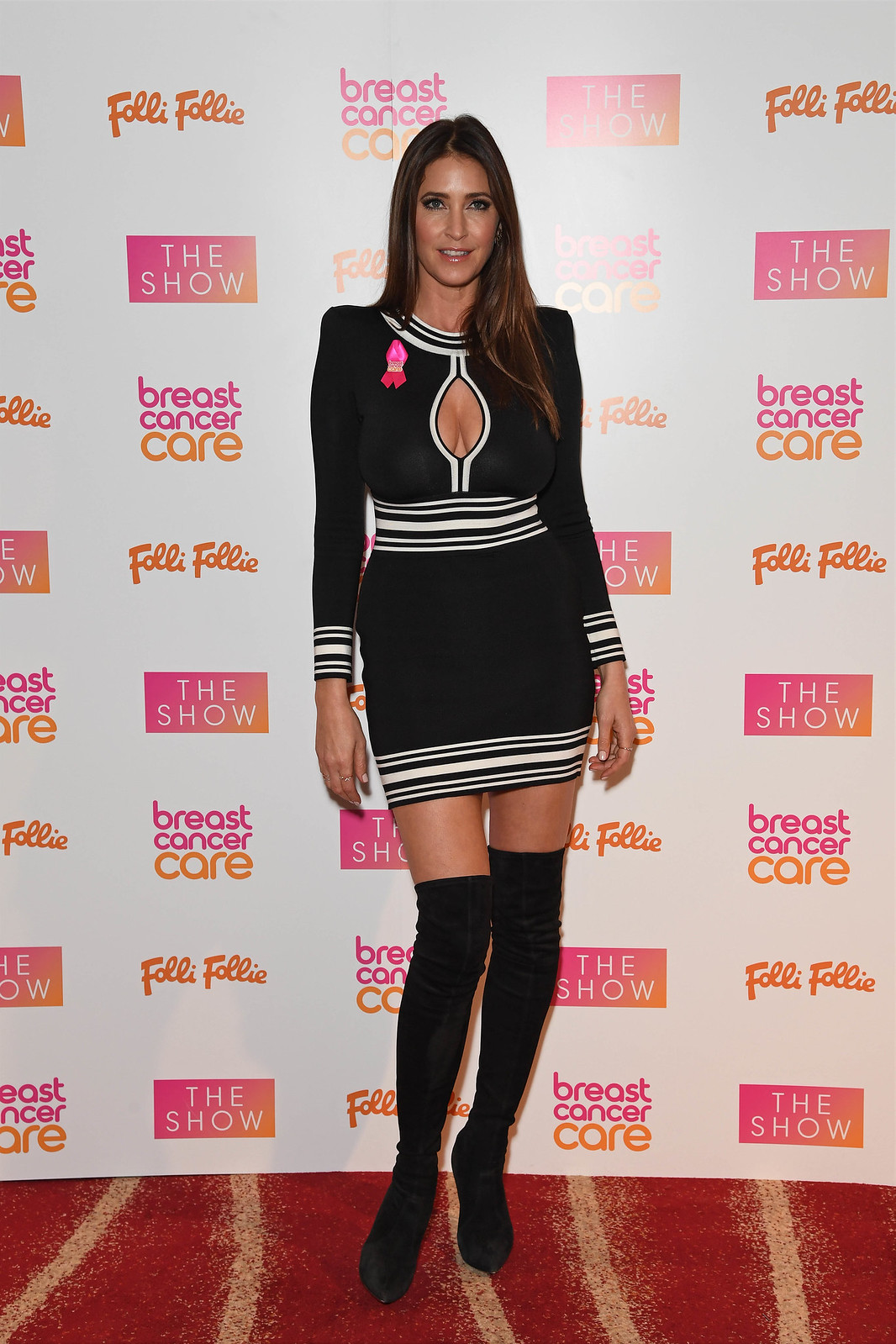The image features Lisa Snowden standing confidently in front of a backdrop filled with repeated logos and text, specifically "Folly Folly," "The Show," and "Breast Cancer Care," indicating a breast cancer awareness event. She has long, dark brown hair cascading past her shoulders and is dressed in a form-fitting black dress with distinct white stripes adorning the neckline, waistline, sleeve ends, and hemline. A pink ribbon, symbolic of breast cancer awareness, is pinned near the top of her chest. The dress is paired with thigh-high black boots that complement her tall, poised stance. She poses with her hands at her sides, her hip slightly tilted to the left, exuding elegance and confidence. The backdrop she stands against is predominantly white with scattered logos, and she is positioned on a red carpet that has lighter tan stripes, adding a touch of glamour to the scene.